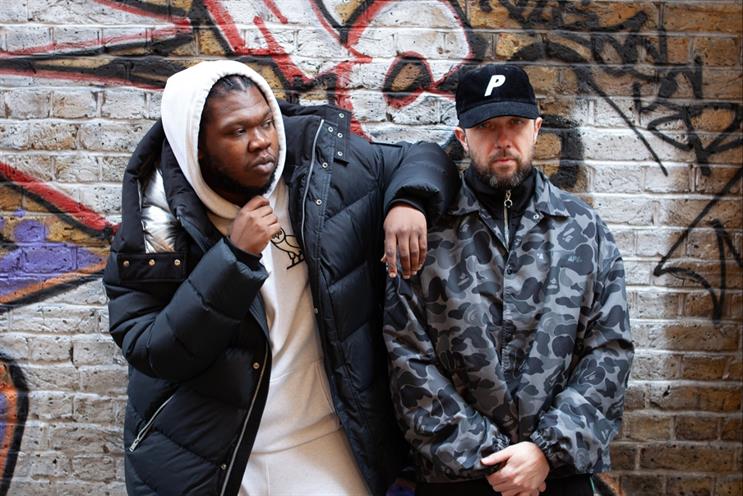The photo captures two men standing close together against a brick wall adorned with extensive graffiti, featuring primarily black, white, red, and purple colors. The man on the left is black African American, wearing a thick puffy black jacket over a white hoodie with the hood up, revealing an owl on the chest. His white sweatpants complement the hoodie, and one arm rests casually on the shoulder of the man beside him while his other hand is under his chin. The man on the right is white, sporting a camo-style army jacket over a black shirt with a zipper. He is wearing a black hat with a white "P" in the center, and his expressionless face is framed by a mustache and beard. His arms are crossed in front of him as he stands slightly more rigid. The close-up shot focuses on their attire and expressions while capturing the richly detailed graffiti behind them, adding a gritty urban backdrop to the scene.